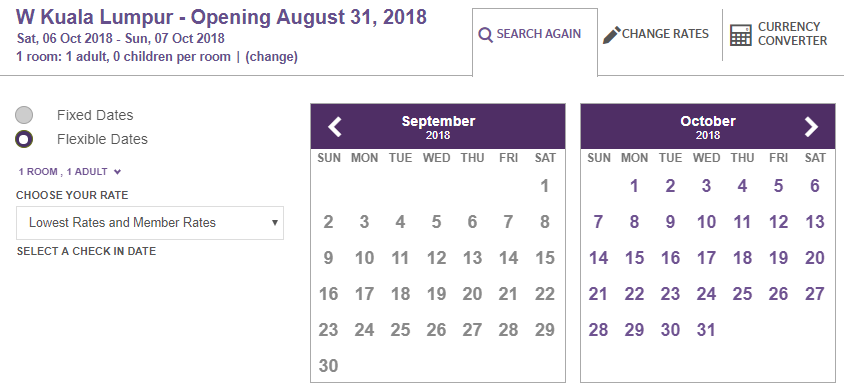The image displays a detailed booking interface from a website, likely related to scheduling a visit to a hotel or similar accommodation in West Kuala Lumpur. At the top left, it is indicated that the opening date for this location is August 31st, 2018. The booking details specify a stay from Saturday, October 6th, 2018 to Sunday, October 7th, 2018, for one room accommodating one adult with no children.

The interface features several functional options, including 'Search Again,' 'Change Rates,' and a 'Currency Converter,' suggesting flexibility and convenience for international users. Two calendars are visible, one for September 2018 (grayed out) and one for October 2018 (highlighted in purple), emphasizing the selected booking dates. Users can choose between 'Fixed Dates' and 'Flexible Dates' for their stay.

There is also a selection menu for room rates, with the current selection being 'Lowest Rates' and 'Member Rates,' indicating a cost-conscious approach. The comprehensive details and tools provided imply that this site caters to both local and international travelers, making it user-friendly for a wide demographic.